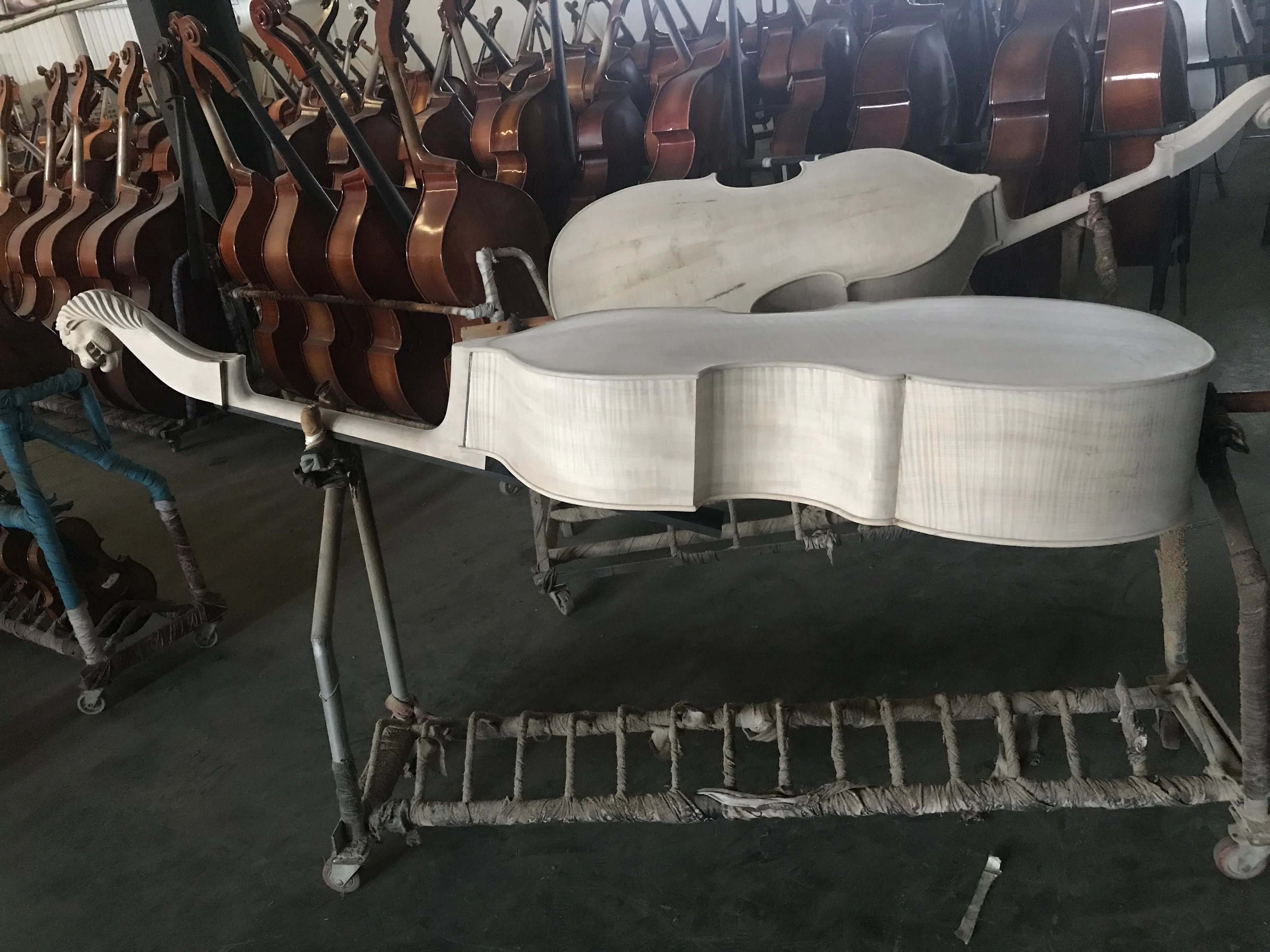The image depicts an indoor scene of a factory or craftsman workshop dedicated to making large string instruments, possibly cellos or basses. In the spacious room, racks upon racks of dark brown finished cellos or basses are neatly lined up in the background. These instruments, standing upright on metal racks, appear to be completely assembled and varnished. At the front right of the image, there is a metal rack holding two unfinished instruments lying face down. These instruments are in a raw, light beige wood state, yet to be painted or varnished. Their handles are intricately carved, possibly resembling a lion's head. The floor of the workshop is a dark gray color, and the overall atmosphere reflects a meticulous, handcrafted process.